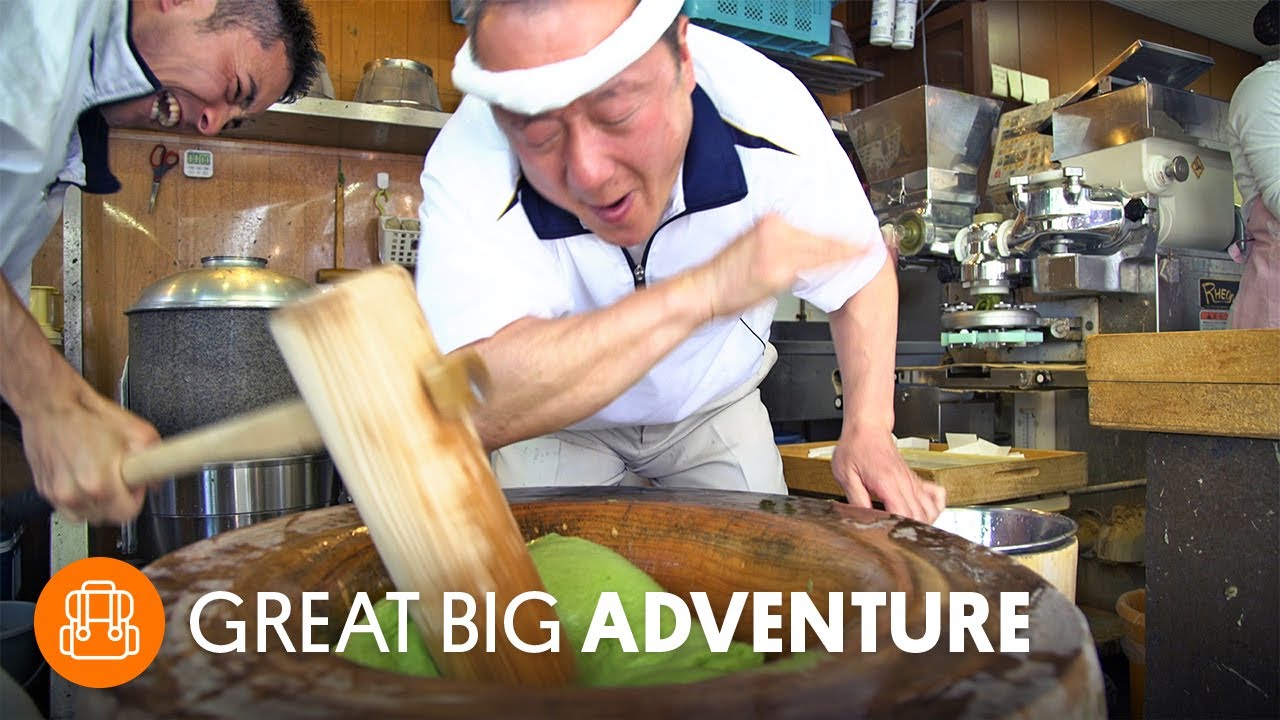This rectangular photograph captures a dynamic scene of two Asian men making rice cakes, with the top and bottom sides of the image being twice as long as the left and right sides. In the bottom left corner, a red circle with a white outline of a rocket ship and the white text "Great Big Story" has been imposed over the photograph. The setting appears to be inside a bustling kitchen or shop. At the center of the image, one man, who has a receding hairline and a white towel wrapped around his head, leans over a large, thick-rimmed wooden bowl. He is wearing a zip-up white shirt with short sleeves and black collar, along with creamy gray pants. His arm is raised, seemingly in the act of pushing or stirring.

Nearby, in the top left corner, another man energetically uses a large wooden mallet to pound a sticky rice mixture inside the bowl. This man, who appears to be in motion with a slightly blurry hand, wears a similar white shirt and looks thrilled, possibly laughing with his mouth open wide. The rice mixture in the bowl might have a green hue, reminiscent of a texture and color similar to guacamole. The lively interaction suggests a moment of shared excitement and concentration as they engage in the traditional rice cake-making process. Surrounding equipment and the energetic expressions on the men's faces convey a busy and joyous atmosphere.